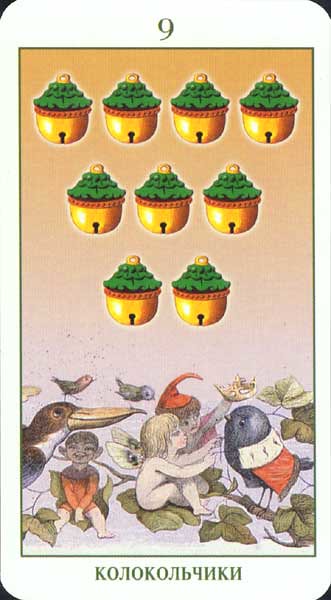This detailed caption describes a colorful and whimsical playing card:

"The card, topped with the number nine, showcases an intricate design. Central to the image are nine bells arrayed in a pyramidal formation: four on top, three in the middle, and two at the bottom. Each bell is detailed with a yellow top resembling a cupcake, adorned with green, tree-like frosting. The bells' bodies are yellow, featuring a dark circular mark at the base and a vertical line extending downward, evoking the appearance of a classic bell. An orange border accentuates the middle of each bell. The background gradient, transitioning from shades of orange, mirrors a sunset. At the card's base, two children interact with a bird: a naked boy and another wearing a red elf-like hat. The bird, larger and more imposing than the children, is a rotund black creature donning a red cape. Additionally, a monkey-like figure is seen crouching in the bottom left corner, adding to the card's fantastical scene."